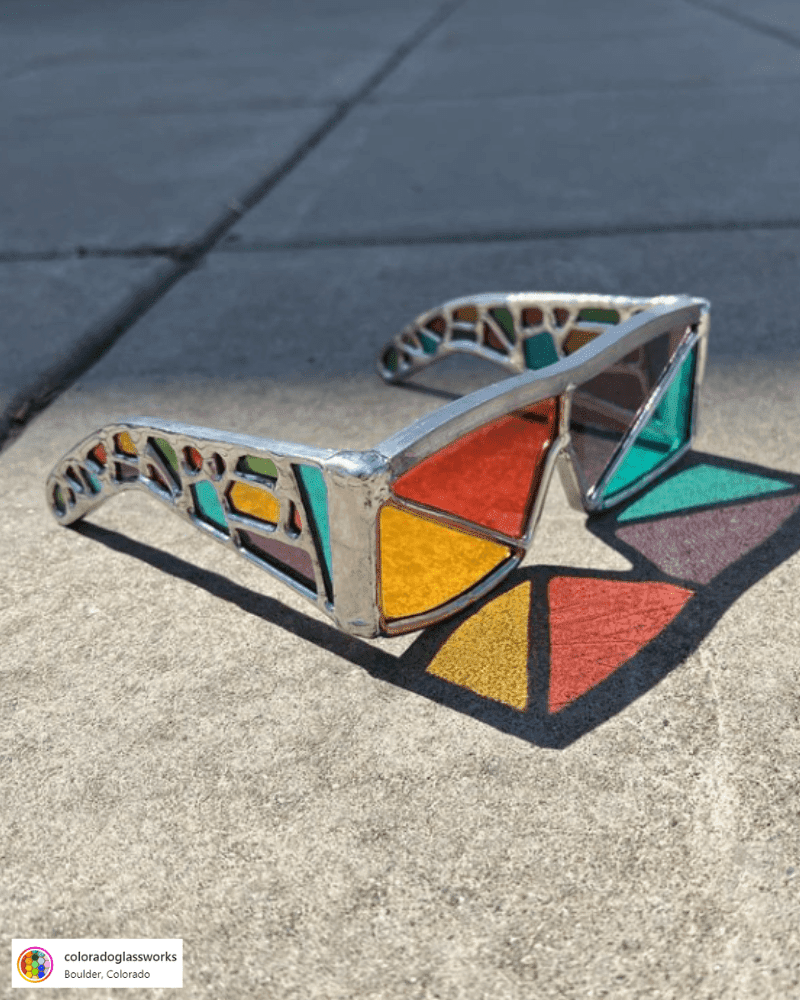This vibrant advertisement-style photograph showcases a pair of handmade, stained glass-inspired glasses resting on a sunlit sidewalk made of grey concrete squares. The glasses feature a sturdy silver metal frame with a distinct art piece feel. The lenses boast a unique four-color combination, with one side displaying yellow and red, and the other side purple and blue, arranged in triangular patterns. The temples are adorned with a mosaic of variously shaped stained glass pieces, including triangles, rectangles, and circles in an array of colors such as aqua, yellow, pink, green, and purple. In the bottom left corner, the image prominently features the logo "Colorado Glassworks, Boulder, Colorado," highlighting the craftsmanship and origin of this striking eyewear.